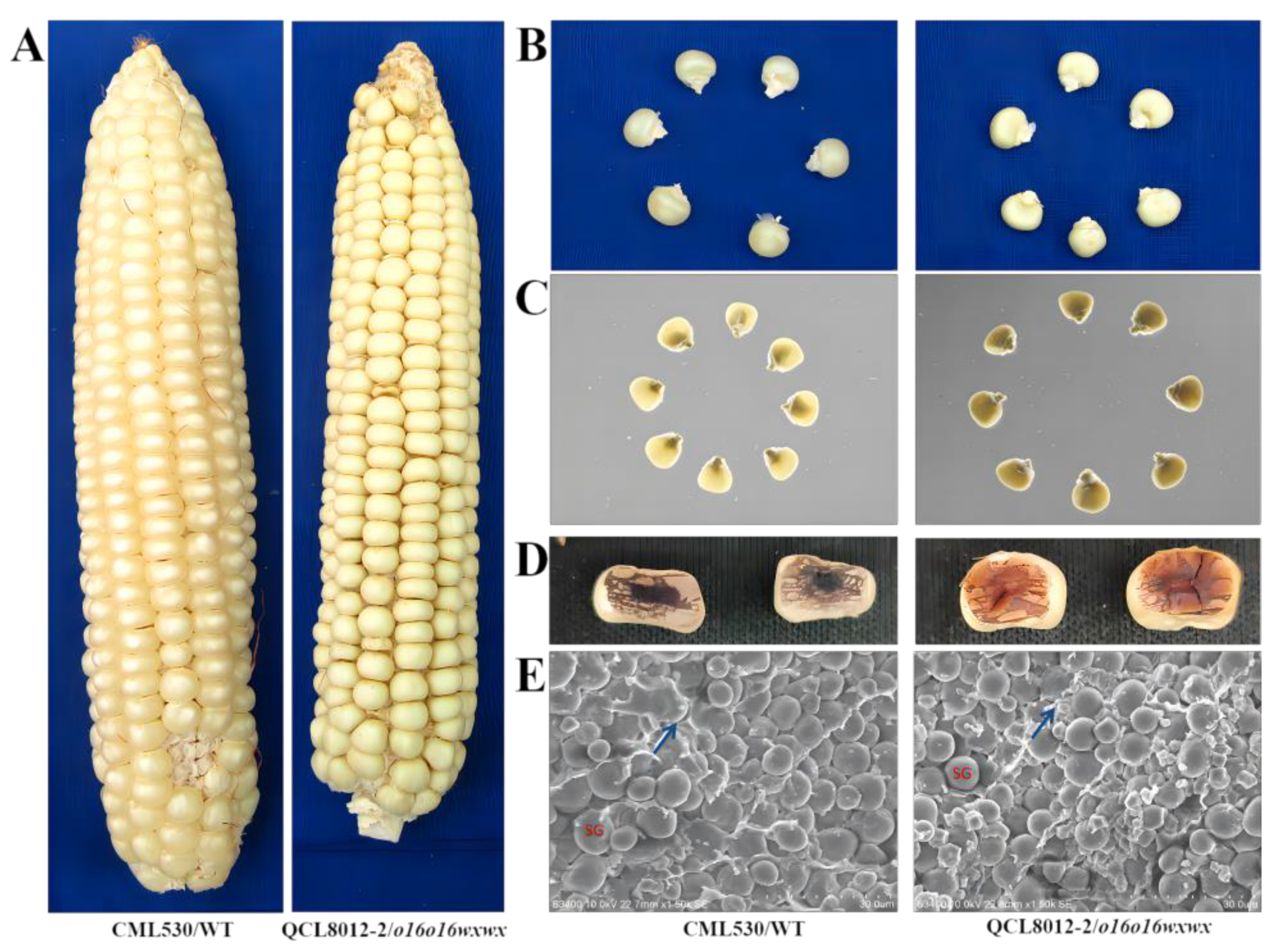The image comprises a detailed series of photographs displaying various aspects of corn and corn kernels. On the left, two images labeled "A" show different ears of yellow corn on the cob, set against a blue background. Below each corn cob, there are specific labels: the first is identified as "CML 530 Wt" and the second as "QCL 8012-2/016/016 WXWX." To the right, the series continues with photographs labeled "B," "C," "D," and "E," each showing successive close-ups of individual corn kernels. Label "B" features kernels arranged in a circular pattern, transitioning to label "C" where the kernels are similarly arranged but set against a gray backdrop. Further close-ups of the kernels are seen in the images labeled "D," possibly showing internal cross-sections or differently magnified views. Finally, images labeled "E" present what appear to be microscopic views of the kernels' surface, depicted as a series of gray spheres with two blue arrows highlighting specific details. Each series illustrates progressively detailed examinations of corn, from whole cobs to intricate microscopic views.